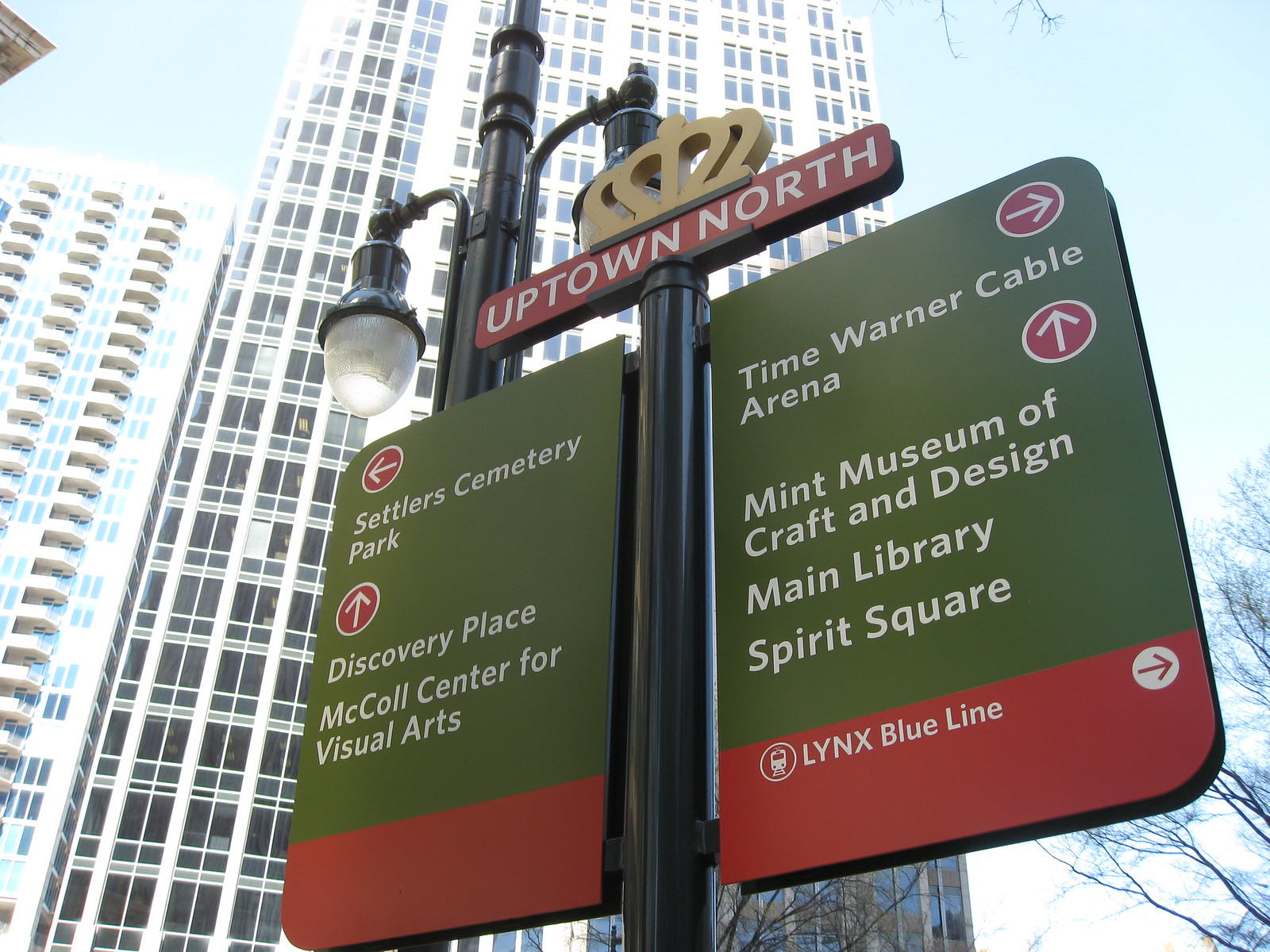This image showcases an outdoor street sign prominently placed in front of a lamppost under a clear, sunny sky. The sign, titled "Uptown North" beneath a crown emblem, provides directional information to various landmarks. The left panel directs to Settlers Cemetery Park, Discovery Place, and McCall Center for Visual Arts, with respective arrows indicating their positions. The right panel guides to the Time Warner Cable Arena, and further ahead to the Mint Museum of Craft and Design, Main Library, and Spirit Square, including information about the Lynx Blue Line on a distinct red background at the bottom. The scene features a towering high-rise building in the background, possibly a residential complex, with another shorter but multi-storied building to the left. A tree's branches partially intrude into the right side of the frame, contributing to the overall urban landscape.